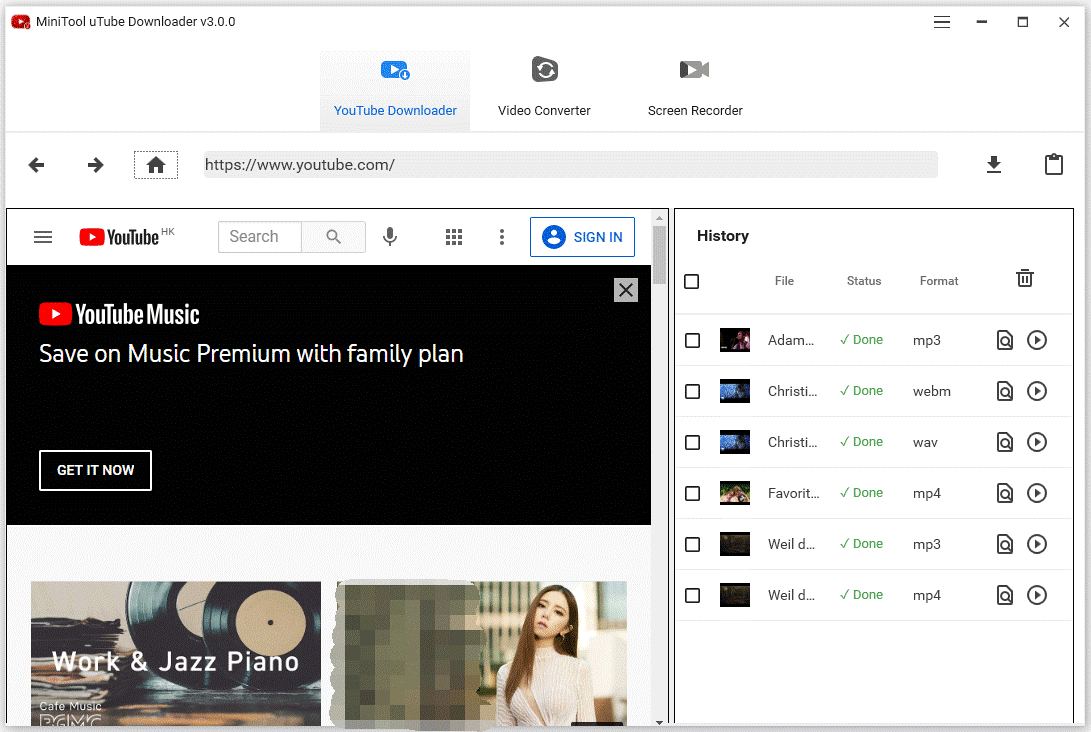In the image, a video downloading interface is prominently displayed, identified as "MiniTool YouTube Downloader Version 3.0.0" at the top left corner alongside the YouTube logo. On the top right of the screen, the typical browser controls – an X for closing, a square for maximizing, and a dash for minimizing – are visible next to a hamburger menu icon.

The interface has three main categories listed in the top menu: "YouTube Downloader," "Video Converter," and "Screen Recorder." Below this menu, the URL bar displays "YouTube.com." The YouTube site is shown beneath with a black screen featuring an advertisement that reads, "Save on Music Premium with Family Plan. Get it now."

To the right of the main video box, there's a vertical rectangular section titled "History," listing six different files with their download statuses marked as "Done." The formats of these files are displayed in sequence from top to bottom: MP3, WebM, WAV, MP4, MP3, and MP4. At the bottom left of the interface, there is a section labeled "Work and Jazz Piano."